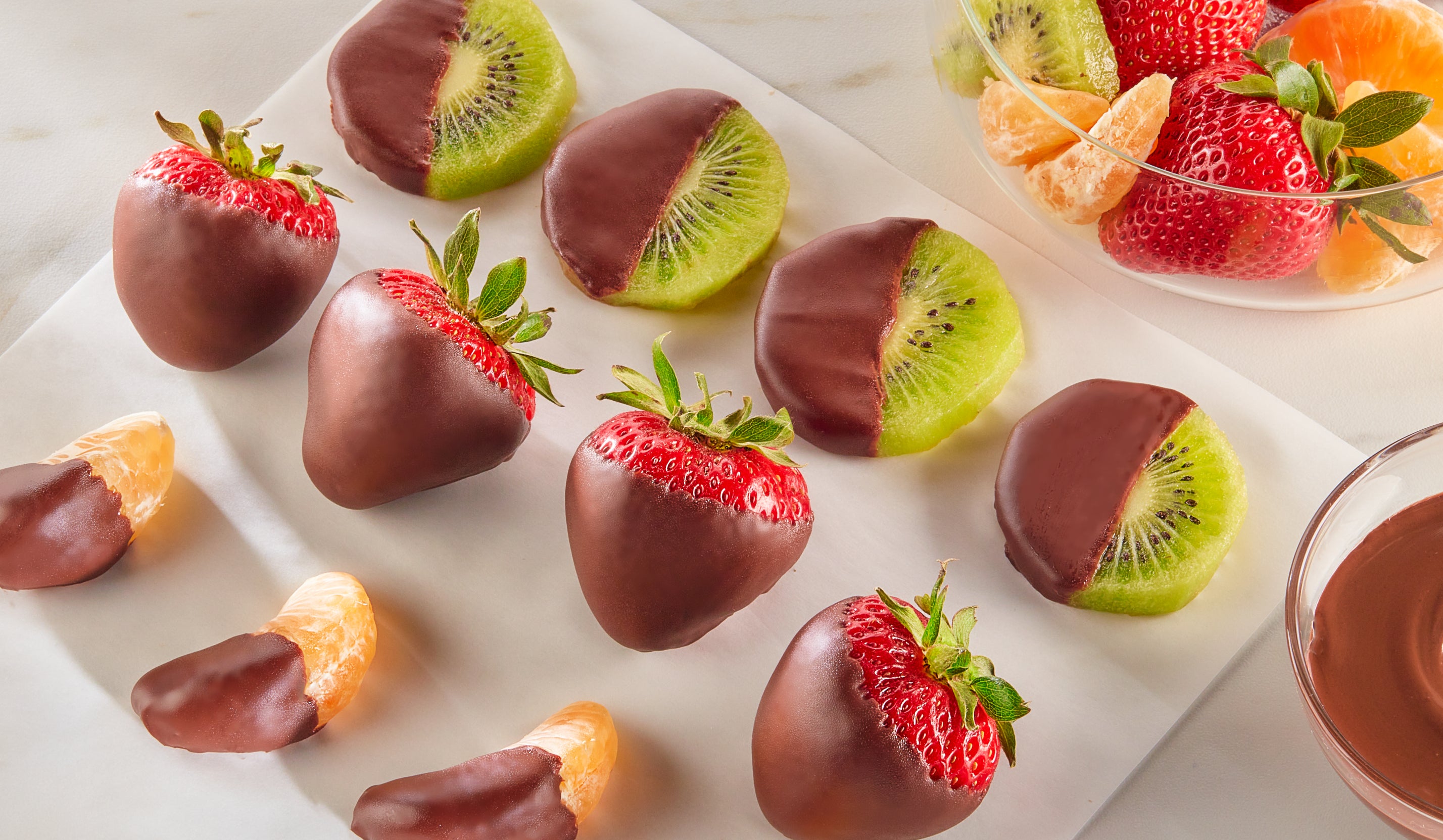This high-definition, professional photo features a beautifully arranged platter of various fruits dipped in chocolate. The main subject is a squared white plate placed on a pristine white marble countertop covered with a sheet of parchment paper. On the plate, there are 12 perfectly organized pieces of chocolate-dipped fruit: four luscious strawberries, four kiwi slices, and four sections of what appears to be clementines, each dipped halfway in creamy milk chocolate.

On the right side of the image, partially cut off, there is a clear glass bowl filled with the same rich chocolate used for dipping. In the upper right portion of the image, another clear bowl brims with fresh, undipped fruit including whole strawberries, sliced kiwis, and clementine sections. The entire scene is brightly lit, highlighting the vibrant colors of the fruit and the glossy sheen of the chocolate, making it look like a photo straight out of a gourmet magazine or a Pinterest board.